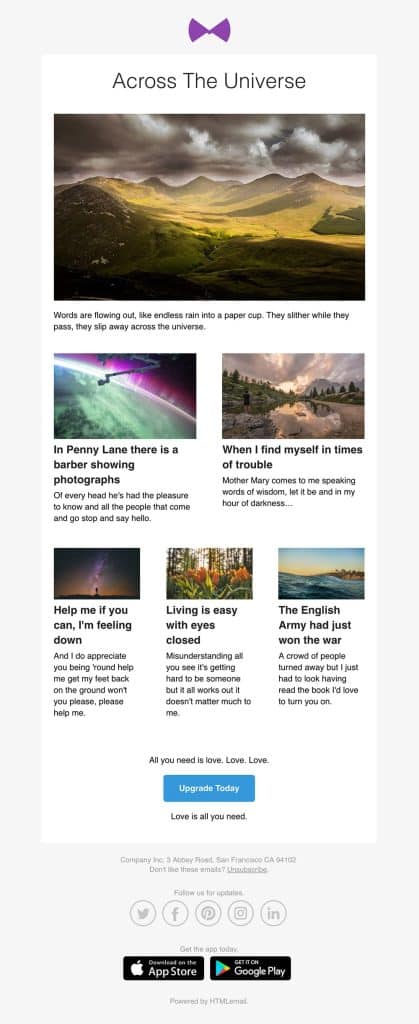In this surreal and symbolic image, words seem to flow endlessly across the expanse of the universe, resembling rain cascading into a paper cup before seeping away. The imagery is vibrant and alive, reminiscent of the iconic lyrics from The Beatles' songs. Headlines drift through the scene, and in a nostalgic corner, a figure in "Penny Lane" displays photographs of various herds he's acquainted with, with people stopping by to greet him. Mother Mary stands in a comforting pose, uttering words of wisdom such as "let it be" to those in their moments of trouble and darkness. The image also captures a plea for assistance with someone feeling down and appreciative of support to get back on their feet. The dreamlike portrayal hints at an easy, almost naive simplicity of life when misunderstood, yet acknowledges the struggle of becoming someone significant. A historical touch appears with the English army's victory, drawing a mix of reactions; a crowd turns away while an intrigued onlooker, who has read the book, feels an irresistible urge to explore further. This visual is an eclectic tapestry of iconic cultural references, woven together to evoke a sense of wonder and introspection.